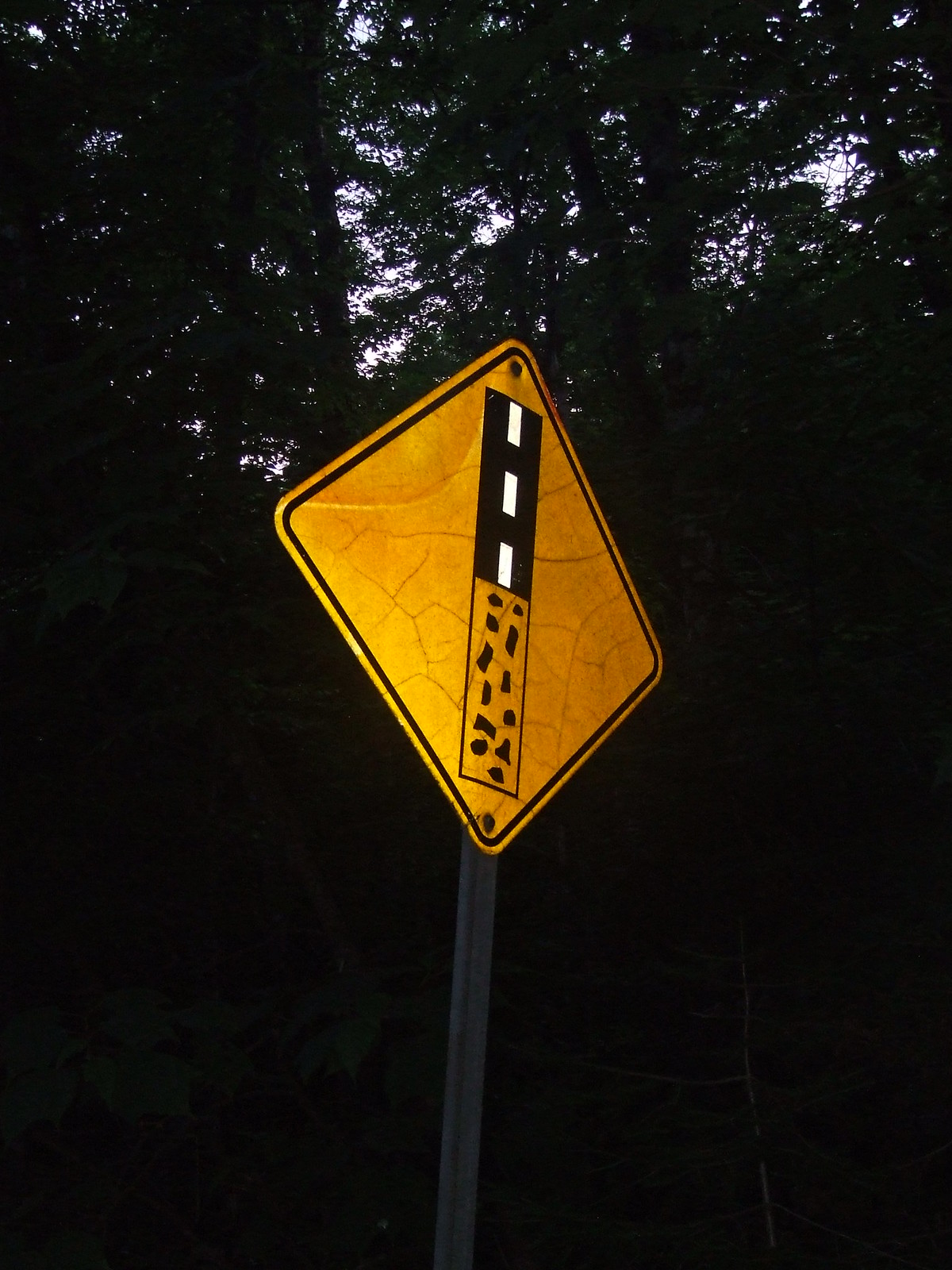In this outdoor image, the sky is predominantly obscured by the dense foliage of numerous trees, rendering the sky a muted white canvas behind the greenery. Central to the scene is a street sign mounted on a grey pole. The sign itself is diamond-shaped with a distinct black border. The interior of the sign features a design of a winding road in contrasting black and white hues against a bright yellow background. The bottom section of the sign displays alternating yellow and black patterns. Surrounding the sign, the lush tree leaves form a rich green backdrop, further encapsulating the natural setting and nearly eclipsing the overcast sky.